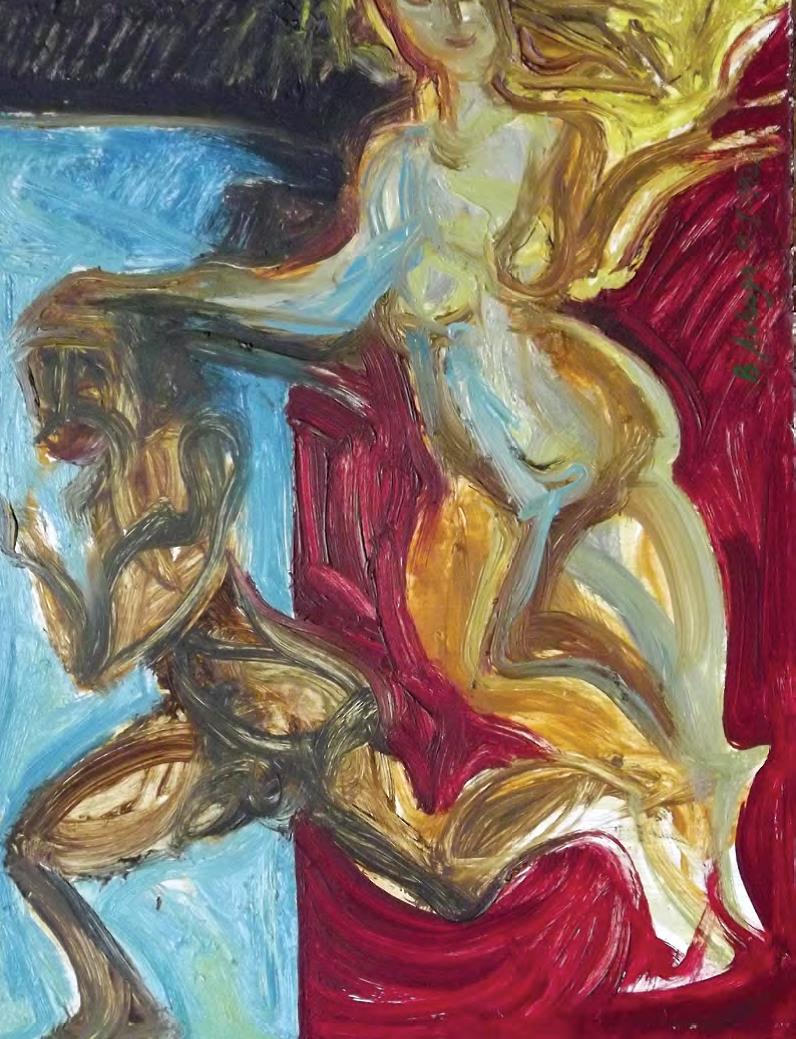This painting, likely acrylic, features a striking juxtaposition of colors and figures, set against a divided background. The upper section of the background is black, transitioning into a deep red on the right and a lighter blue on the left, with a distinct straight border separating these hues. The artwork depicts two figures painted with a palette of white, tan, yellow, brown, and black. A taller, golden-hued woman stands prominently on the right side, her hair flowing behind her, with her hand placed delicately on the head of a shorter figure. This smaller person, likely a man, appears to be running towards the left, his form rendered in darker tones of brown and black. The overall style of the painting leans toward an abstract or impressionist feel, emphasizing form and movement over realistic detail. This expressive piece, devoid of any text, evokes a scene that could easily be found in an art show or museum, inviting viewers to interpret the dynamic interaction between the two figures.